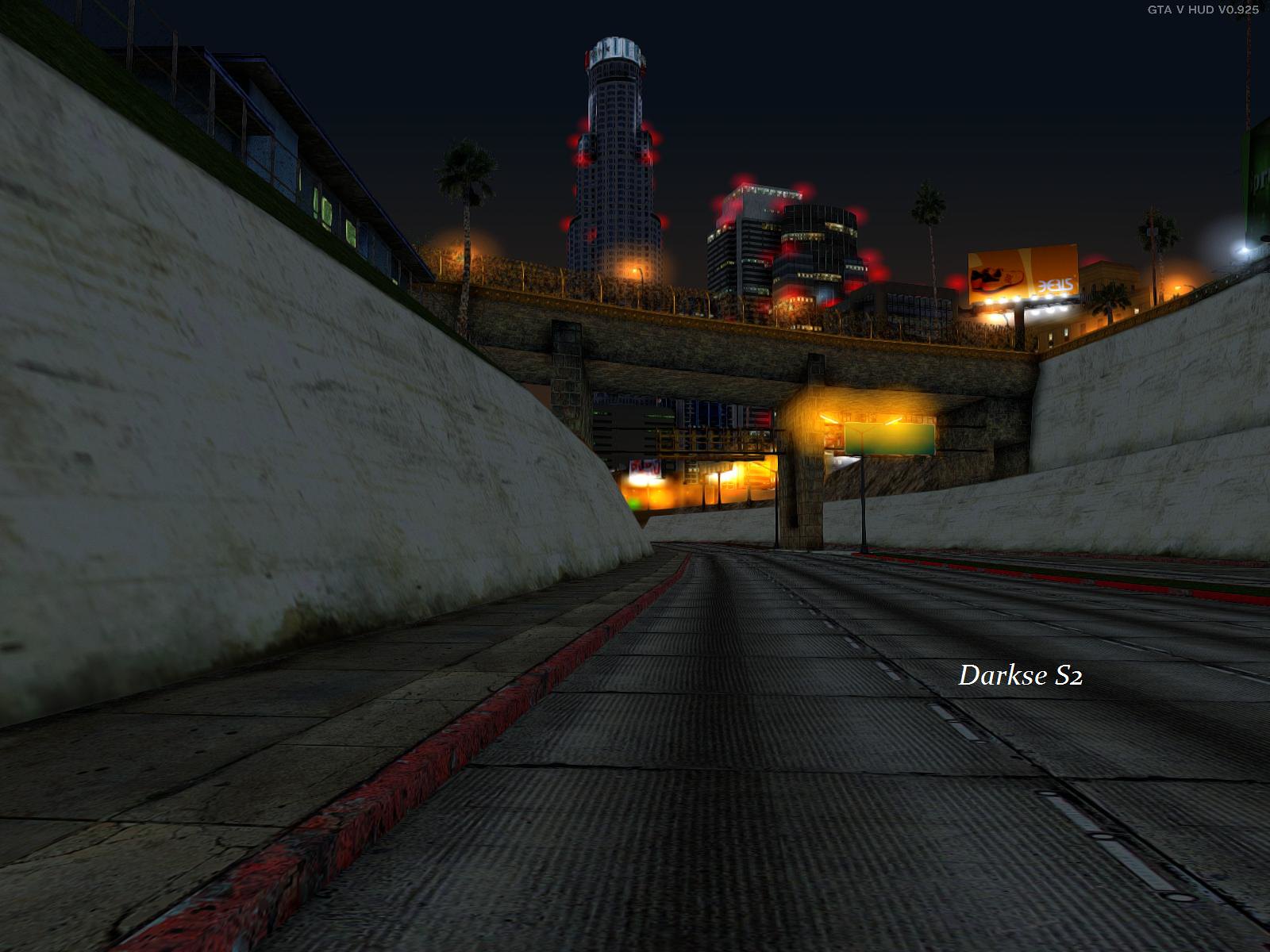This animated image, reminiscent of a scene from a game set in Los Angeles, depicts a concrete road nestled within an urban canyon, flanked by tall concrete barriers on either side. The road, marked by white dashed lines and red-painted curbs, is visibly cracked and descended below the street level, leading towards a small, stone-like bridge with an ornate yellow caged top. Above the bridge, the night sky stretches over tall buildings crowned with red and bright street lights. To the right, yellow street lights illuminate the scene in the background. Palm trees punctuate the cityscape, and a billboard adds to the urban glow. The perspective from the front of a car emphasizes the journey underneath the bridge, immersing the viewer in the nocturnal, bustling ambiance of an inner-city road.